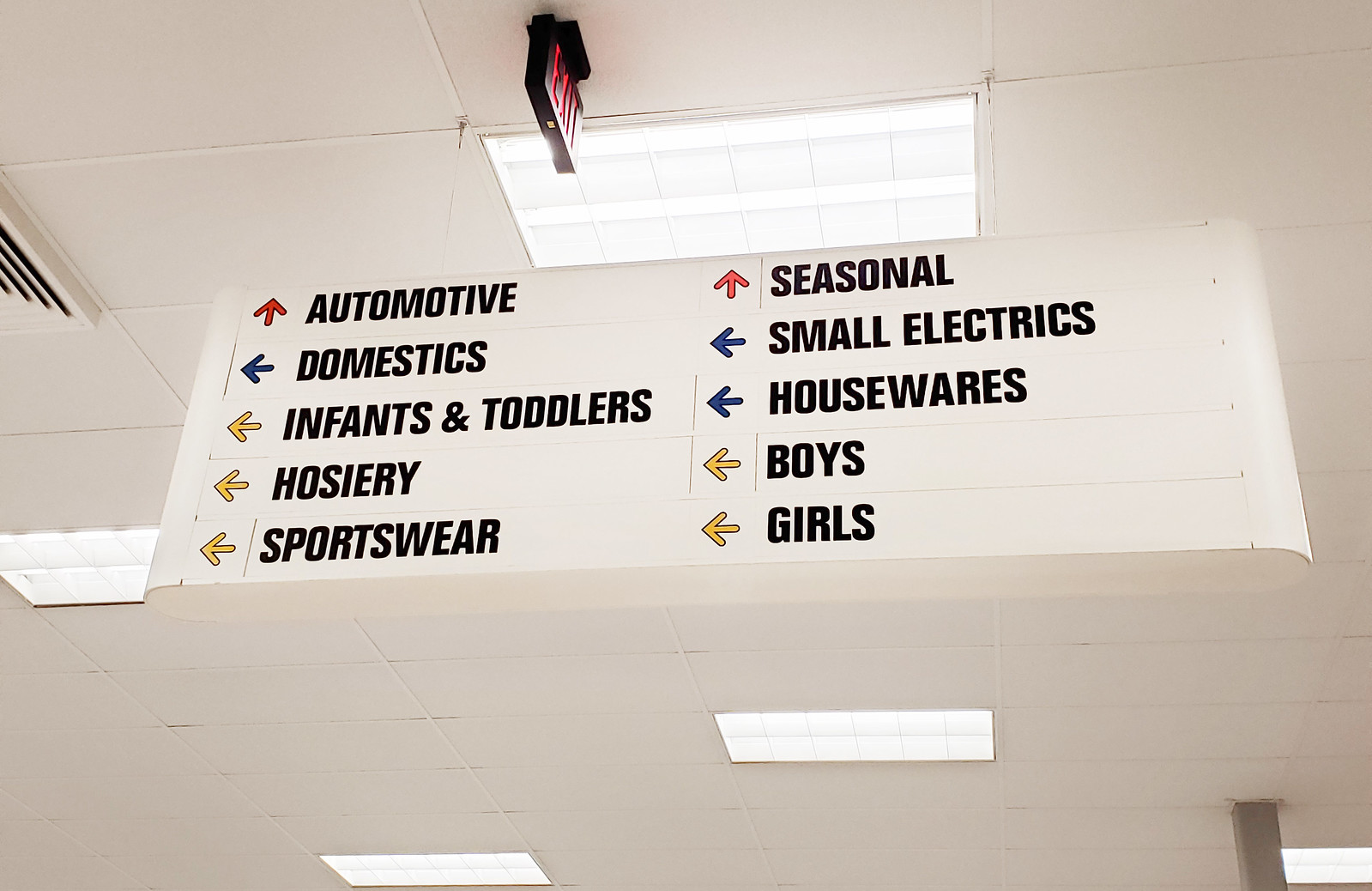The image depicts a horizontal, realistic photograph of a store's ceiling, featuring a white drop cloth ceiling supported by white tracks and illuminated by white overhead lights. A white sign with black text and colored arrows is prominently displayed, indicating various sections within the store. The sign consists of two columns:

- In the left column: 
  - A red arrow pointing up labels the "Automotive" section.
  - A blue arrow pointing left directs to "Domestics."
  - Three yellow arrows pointing left guide towards "Infants and Toddlers," "Hosiery," and "Sportswear."

- In the right column: 
  - A red arrow pointing up marks the "Seasonal" section.
  - Two blue arrows pointing left indicate "Small Electronics" and "Hosiery."
  - Two yellow arrows pointing left lead to "Boys" and "Girls."

This detailed signage suggests it is from a department store with diverse sections including clothing, electronics, and seasonal items.